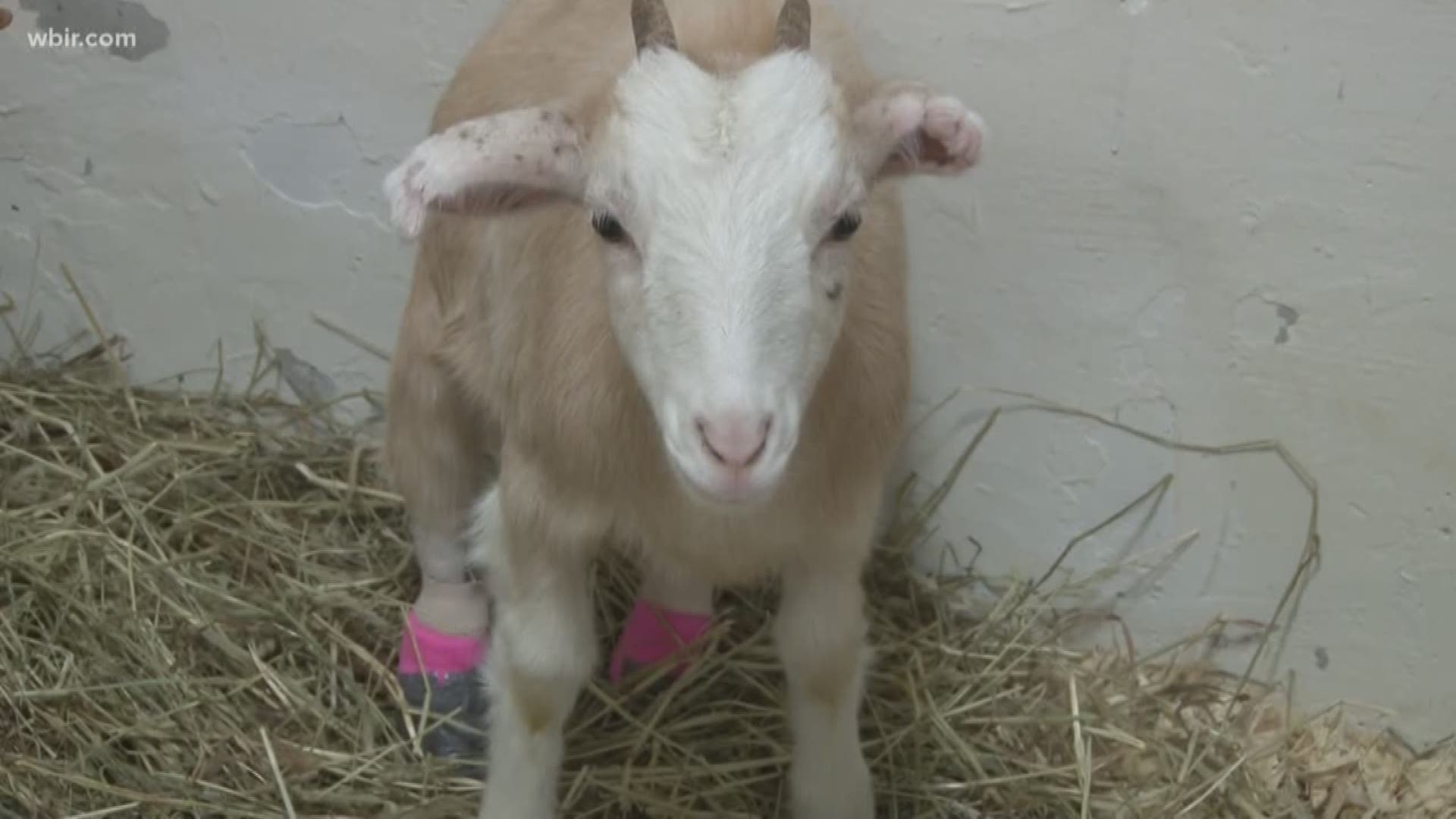The image showcases a young, light brown goat with a mostly white face, interspersed with mottled brown patches. It has distinctive gray horns and ears that stick out to the sides. The goat's back hooves are notably covered in what appears to be hot pink, resembling either children's shoes or protective socks. It is standing on a bed of straw against a white cement or plaster wall, giving the impression it could be located at a petting zoo, farm, or backyard. The goat, with its pink nose and dark brown eyes, gazes directly into the camera. In the upper left corner of the image is a watermark that reads "WBIR.com".